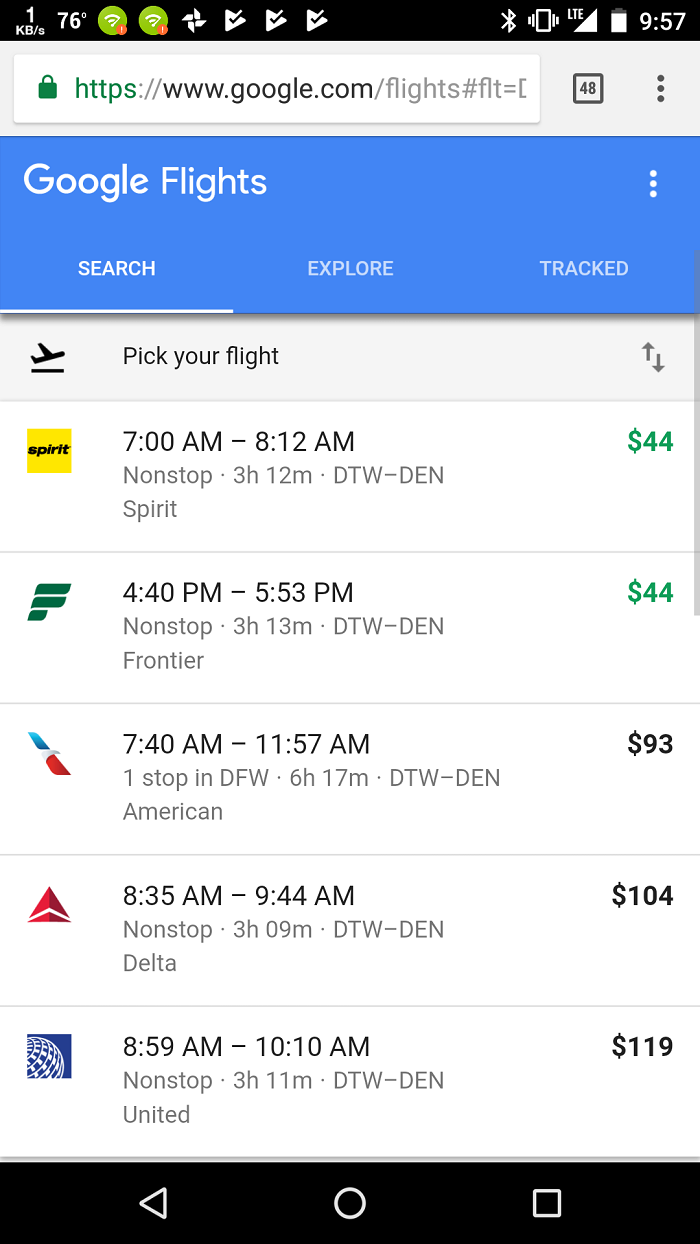The screenshot depicts a detailed interface of a smartphone with an active Google Flights search. At the top, the status bar is set against a black background displaying various standard smartphone icons in white, including a number showing 1 KB/s, green illuminated wireless icons, a white pinwheel design, and three angled triangles with check marks. On the right side of the status bar, standard icons like Bluetooth, LTE network signal, a mostly full battery icon, and the time (9:57) are visible.

Beneath the status bar is a white rectangular data entry or search box displaying the URL www.google.com. Adjacent to this box, there is a small square with the number 48 in it, followed by three vertical dots symbolizing additional settings options.

Below this, a wide blue title bar labeled "Google Flights" is present, featuring three sub-options: Search, Explore, and Track, with "Search" currently selected. Another set of three vertical dots is located on the far right side of this bar for further settings.

The section below is headed with "Pick your flight," accompanied by a small icon of a plane taking off. To the right of this header are up and down arrows for navigation. Five rows of flight options are displayed underneath. 

Each row contains:
1. Airline logos on the far left: starting with Spirit, followed by Frontier, American, Delta, and United.
2. In the center, detailed travel information such as travel times, flight durations, and whether the flights are non-stop or connecting, alongside airport codes.
3. On the far right, flight prices are listed, with the first two rows highlighted in green to indicate the lowest prices.

The interface provides a comprehensive overview, enabling users to select and compare flights efficiently based on their preferences.